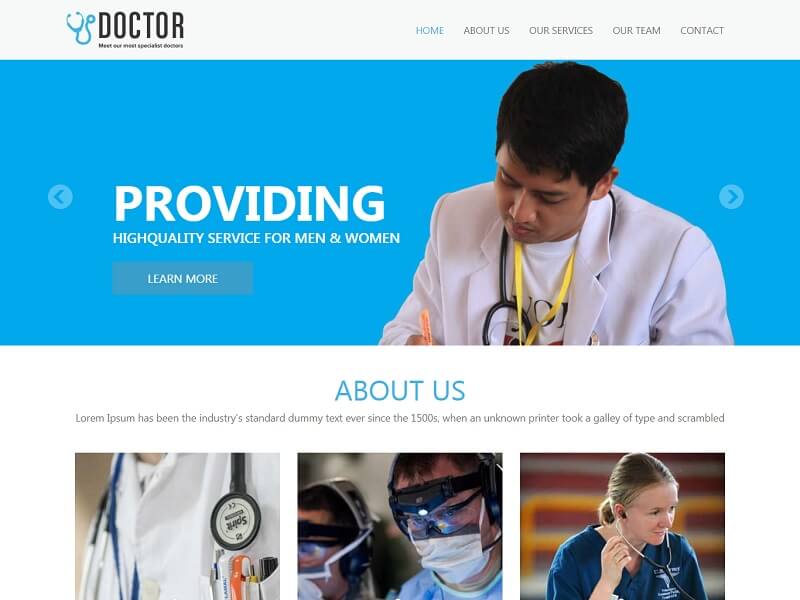The webpage features a clean, professional design centered around medical services. At the top left of the page, there's text displaying "Top Doctor" against a white banner. Adjacent to this on the right is a navigation bar with options labeled: Home, About Us, Our Services, Our Team, and Contact. To the left of the "Top Doctor" text, there's a small blue stethoscope illustration.

Below the banner is a large image with a blue background. Prominently displayed in the center-left of this image are the words "Providing" in bold white letters, followed by "High-Quality Service for Men and Women." Beneath these statements, there is a "Learn More" button. The right side of the image features a doctor with brown skin and black hair, wearing a white doctor's coat, looking down as he writes something on a notepad.

Further down the page, there's an "About Us" section, indicated by blue text against a white background. The section begins with placeholder text, starting with "Lorem Ipsum" and traditionally used as industry-standard dummy text since the 1500s. Below the text are three images: 

1. A doctor's coat hanging up.
2. Two doctors, one with fair skin, dark hair, wearing a face mask, glasses, and black headgear; the second person's face is mostly cut off but appears to be wearing similar headgear.
3. A fair-skinned woman with dark blonde hair, wearing a blue nurse's t-shirt and a black stethoscope.